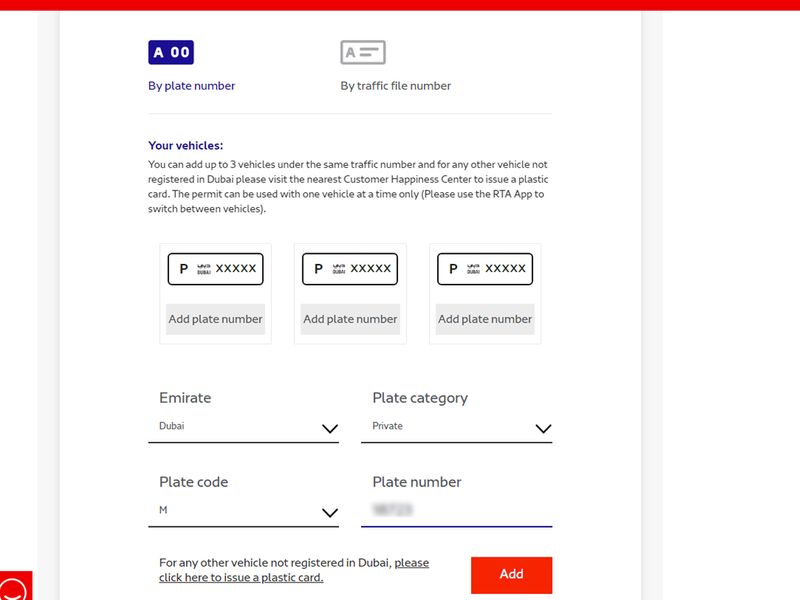This is a detailed screenshot of a user interface for managing vehicle permits. In the bottom left corner, there is a red icon featuring a half-circle and a line resembling a smile. The main section of the page displays a computer-generated document with shadowed edges, giving it a realistic paper-like appearance.

In the top left corner of this document, there is a blue box labeled "A00," under which the words "by plate number" are highlighted. To the right, highlighted in gray, is an option with the letter "A" flanked by two lines, labeled "by traffic file number." 

Beneath these options, the section titled "Your Vehicles" explains that users can add up to three vehicles under the same traffic number. It also mentions that for vehicles not registered in Dubai, users should visit the nearest customer happiness center to issue a plastic card. The permit can be used with one vehicle at a time, and users are directed to use the RTA app to switch between vehicles (this instruction is enclosed in parentheses).

Following this, there are three smaller boxes, each containing a dark blue rectangle outlined with a "P" and some unreadable text. Five X's are positioned to the right of these boxes. Below each box, there is a gray button labeled "add plate number."

Further down, there are four categories for vehicle details:
1. **Emirate**: A drop-down menu with "Dubai" selected.
2. **Plate Category**: A drop-down menu with "private" selected.
3. **Plate Code**: A drop-down menu with "M" selected.
4. **Plate Number**: The plate number is obscured.

Lastly, another notice prompts users to click a link to issue a plastic card for any vehicle not registered in Dubai. An orange button labeled "Add" is positioned at the bottom.